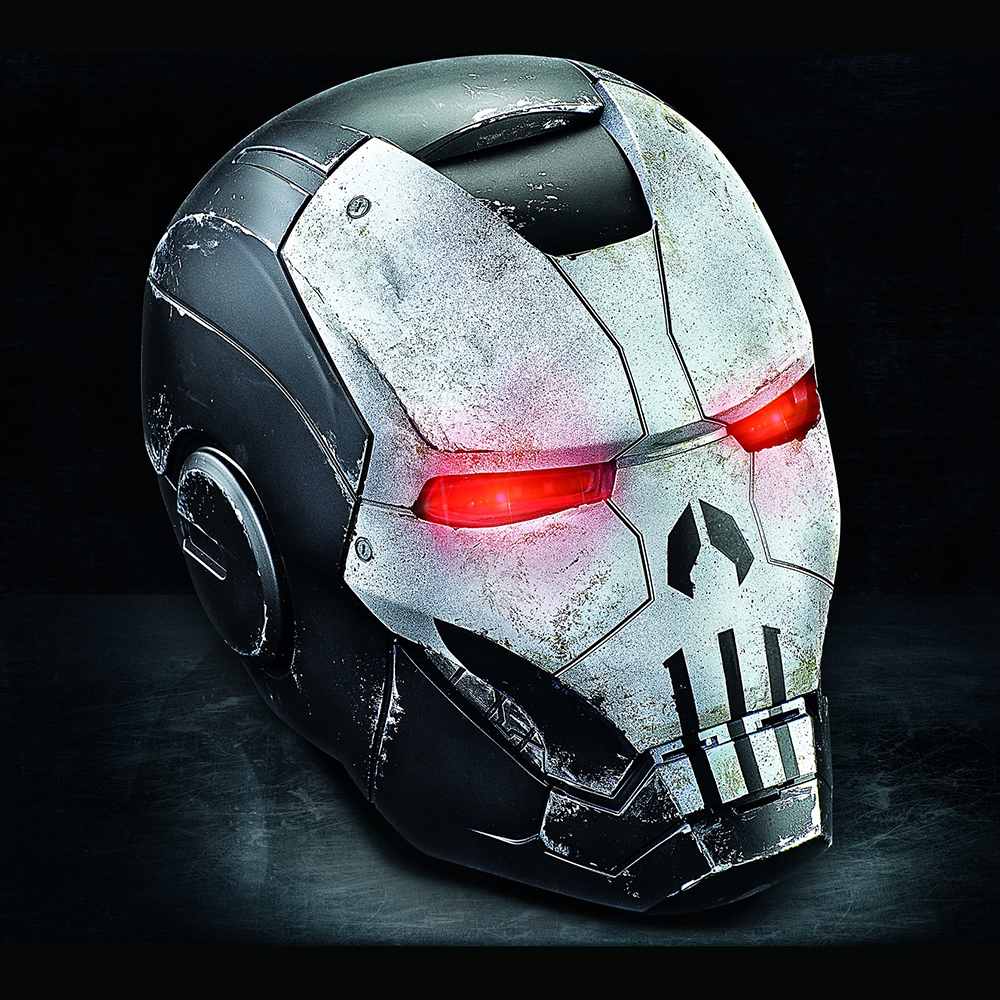The image is a digital artwork resembling the helmet of Iron Man. The mask, inspired by Iron Man, is prominently featured in the foreground, resting on a metallic, black marbleized surface. It has an overall distressed appearance, suggesting signs of wear and battle, with scuffing and etchings particularly noticeable on the left side. The mask itself is predominantly black around the top of the head, ear areas, and jawline, while the front face plate is a light gray or white, painted to resemble a skull. The skull's details include black coloring around the nose and a black skull line. Four screws secure the face plate. The most striking feature is its eyes, which glow a vibrant red, adding a menacing touch to the design. The background of the image is entirely black, enhancing the dramatic contrast with the helmet’s colors.